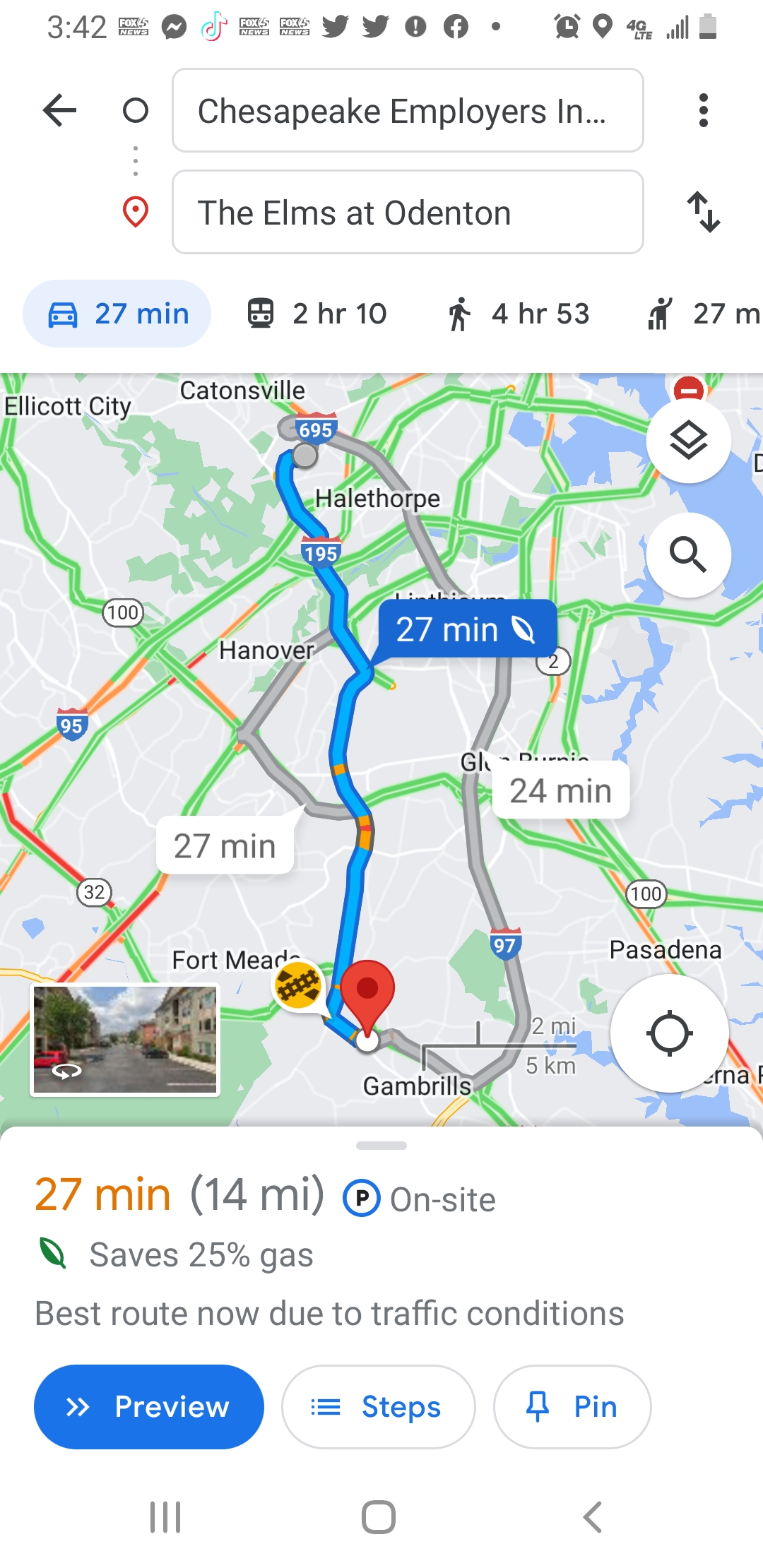A smartphone screenshot displaying a navigation app, closely resembling Google Maps, occupies the center of the image. The smartphone's interface includes a status bar at the top left corner, displaying the time and several app icons indicating active background applications, including Messenger, TikTok, and two instances of Twitter.

In the navigation app, Chesapeake Employers is marked as the starting point, while The Elms of Oddington is designated as the destination. The map highlights three suggested routes with estimated travel times of 27 minutes, 27 minutes, and 24 minutes respectively. The destination is indicated with a distinct icon. Additionally, a notification at the bottom of the screen notes potential fuel savings of 25% for this journey.